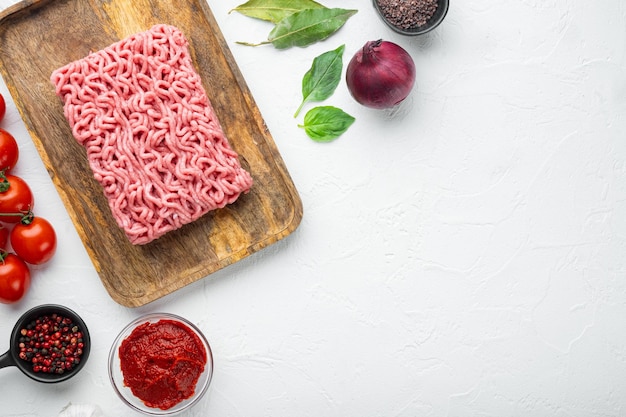The image shows a food preparation area, likely for an Italian dish, set on a clean white countertop. Centered on a wooden cutting board is a rectangular portion of ground beef, approximately a pound in weight. To the left of the cutting board, a cluster of small cherry tomatoes adds a pop of red color. Nearby, a measuring cup brims with a mix of red and black seeds, possibly peppercorns or pomegranate seeds. A small glass bowl beside it contains a rich tomato paste. Scattered around the board are fresh basil leaves and a red onion, enhancing the vibrant, fresh aesthetic of the ingredients. Another small container at the edge of the image holds dark spices or seeds, possibly peppercorns. The professional photograph, suited for a cookbook, captures each element in a crisp, detailed manner, emphasizing their textures and colors against the bright white background.